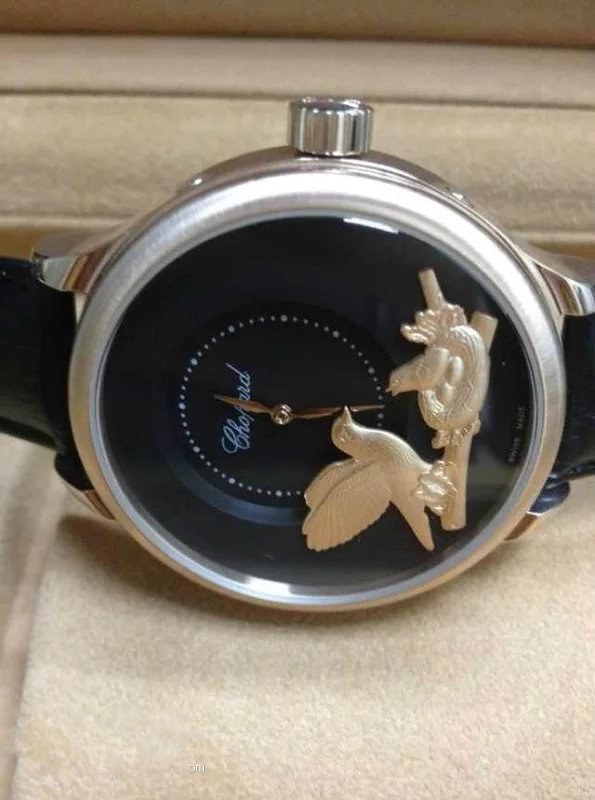This close-up photograph showcases a wristwatch lying on its side against a beige carpet or thick fabric. The watch features a matte black or dark blue face with a recessed, beveled area adorned with small white dots in place of numbers. The face of the watch is oriented slightly towards the viewer, with the top to the left, and the black band extending out of view on both sides. At the center of the watch face, cursive text that might read "Chopard" is subtly inscribed, though it is somewhat hard to decipher.

Dominating the lower section of the watch face is an intricate gold-colored design depicting a mother bird, possibly a pigeon, standing on a branch with its wings uplifted. In front of the adult bird is a nest containing two oblong-shaped eggs and a baby bird looking up at its parent. The silver-toned watch frame complements its traditional, non-digital aesthetic, characterized by sculpted metallic hands—likely silver or gold—that point towards the top and bottom right, framing the tender family scene.